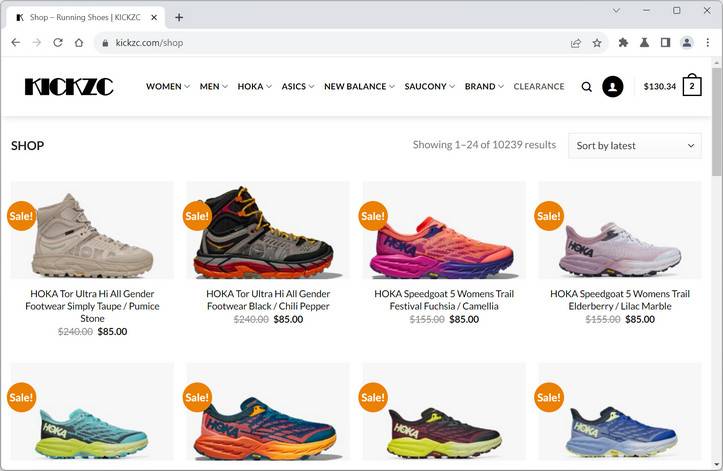The captioned image displays the homepage of "Kickz," an online retailer specializing in athletic footwear and sneakers. The logo is prominently positioned in the upper left corner of the webpage, accompanied by a navigation menu to the right. This menu features categories such as Women, Men, Hoka, Asics, New Balance, South Sydney Brand, and Clearance. Additionally, there is a magnifying glass icon, likely for search functionality, an account icon represented by a circle with a person's image, and a shopping bag icon with a '2,' indicating items already in the cart.

Below the navigation bar, the page showcases two rows of four brightly colored athletic shoes each. The top row includes:
1. Hoka Tour Ultra High All-Gender Footwear in Taupo Pumice.
2. The same model in Black and Chili Pepper.
3. Hoka Speed Goat Five Women's Trail Festival in Fuchsia Carmela, featuring a vibrant, rainbow-like design.
4. The same shoe in a more subdued Elderberry Lilac Marble colorway.

In the second row, the shoe names are not visible, but they display the following color schemes:
1. Turquoise and lemon yellow.
2. A shoe with gradient hues between orange and purple.
3. A shoe in yellow and deep purple.
4. A shoe in various shades of blue.